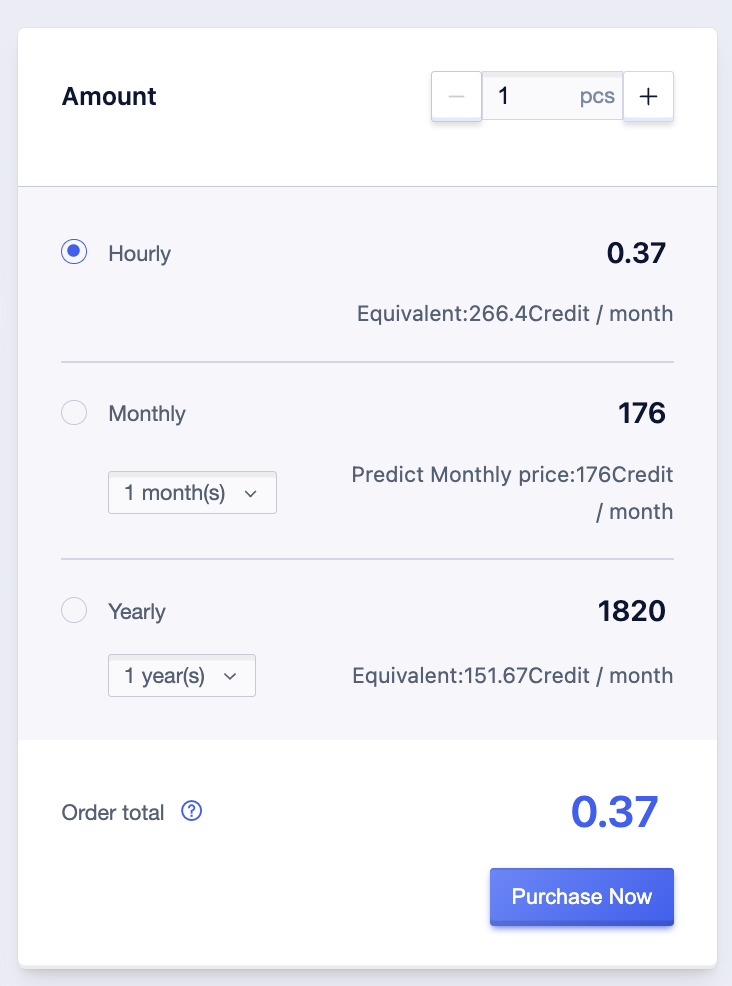The screen displayed is a product purchasing interface with a predominantly white background contrasted by a gray border and various sectional demarcations. At the top, a quantity selector is present, featuring a mount label and adjacent controls for adjusting the item count. A minus button (-) and a plus button (+) flank a central display showing "1 PCS," indicating a single piece, with the ability to increment or decrement the count.

Directly below, two radio buttons offer different pricing models. The first, labeled "Hourly," is selected and shows a rate of 0.37 credits per hour, with a subtext indicating an equivalent monthly cost of 266.4 credits. The second radio button, labeled "Monthly," remains unselected. Beneath it, a dropdown menu displays "1 month(s)," priced at 176 credits, and the predicted monthly price is confirmed as 176 credits/month.

A third pricing option, labeled "Yearly," shows another radio button that is also unselected. Below it, a dropdown option states "1 year(s)," with a corresponding total of 1820 credits. The equivalent monthly cost is calculated to be 151.67 credits/month.

At the bottom of the interface, an "Order Total" section prominently displays the current cost of 0.37 credits in bold blue text. Below this, a call-to-action button, marked "Purchase Now," invites the user to finalize the transaction.